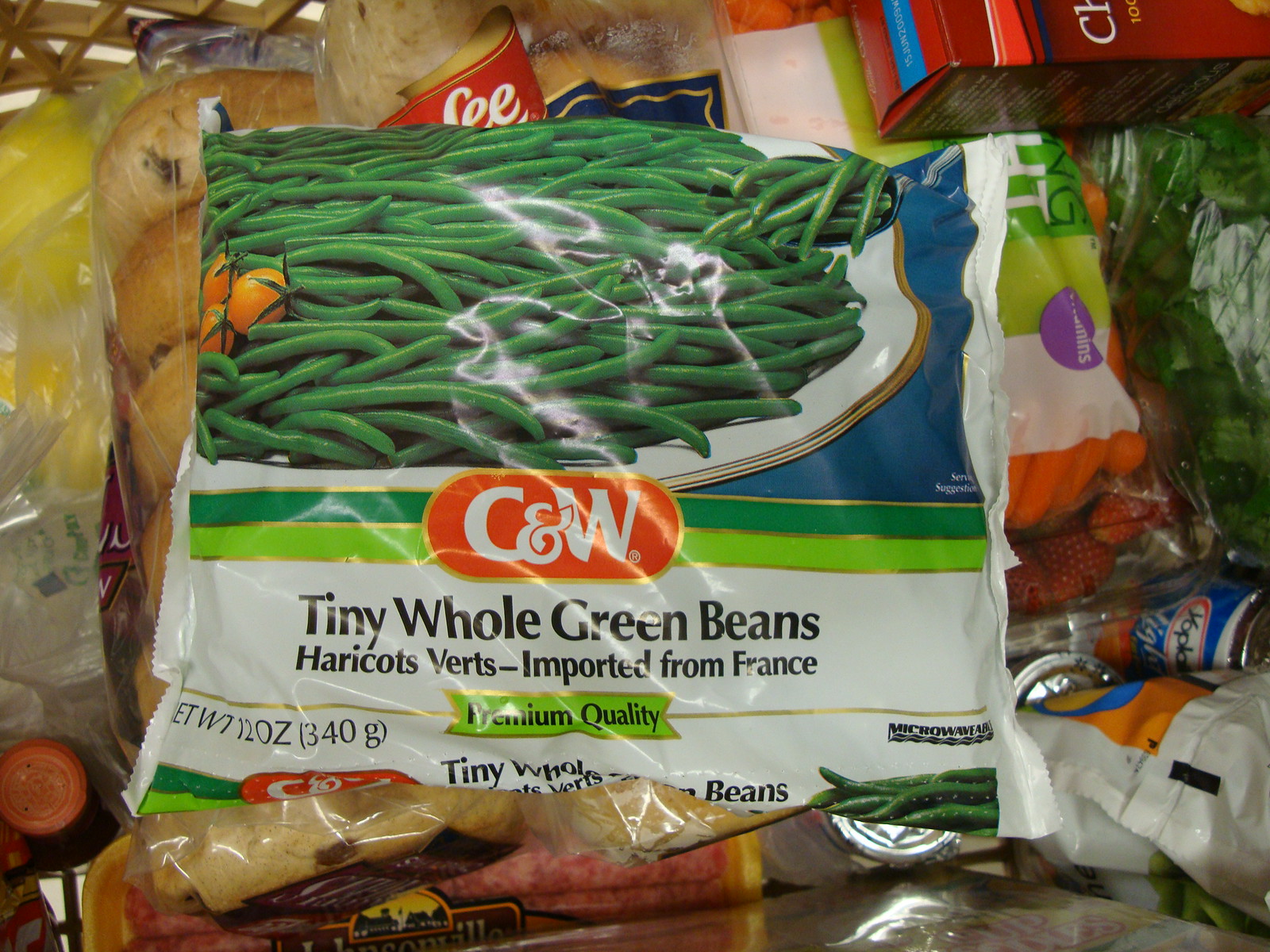The rectangular image, oriented horizontally, predominantly features a bag of frozen tiny whole green beans from C&W, boasting premium quality and imported from France. The package design includes an image of green beans on a white plate against a blue background, adorned with some cherry tomatoes to the left. The C&W logo is prominently displayed in white on a red oval set against a band of dark and light green. The label, “tiny whole green beans, haricot verts,” is printed in black on a white background, alongside a light green ribbon that states "premium quality" in black, bordered with a gold edge. The net weight of 12 ounces (340g) is noted in black text, with "microwavable" indicated on the right. This primary visual element is set against a backdrop of assorted groceries, including a container of carrots, a Sara Lee bread bag (evident from the partial text "L-E-E"), a package of possibly raisin-topped bagels, a Yoplait yogurt cup on the right, and assorted other items such as soda, yogurt, crackers, and potentially some sausages.